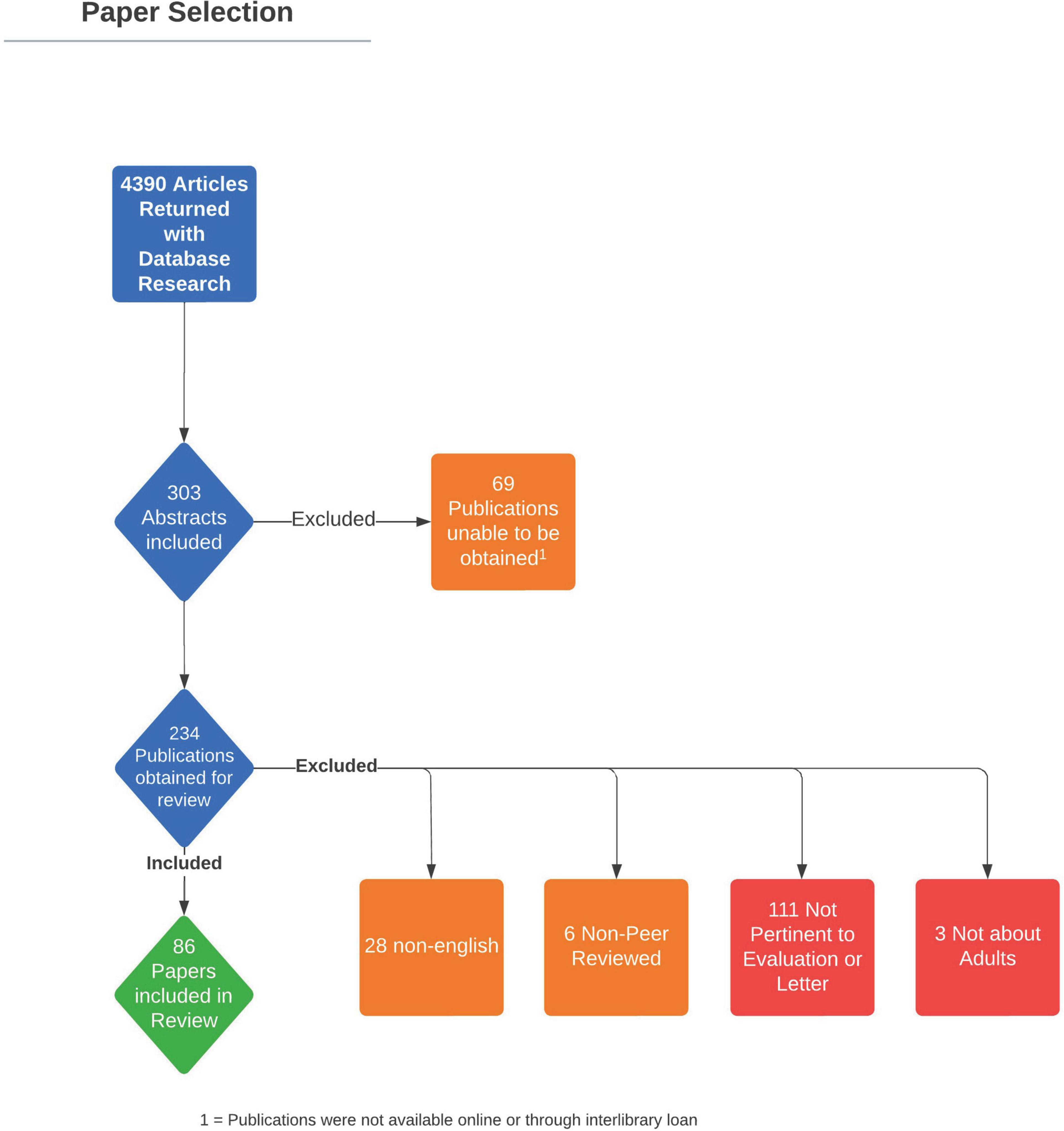This image is a detailed flowchart entitled "Paper Selection," shaped in an L configuration. Starting at the top left, the process begins with a black text label "Paper Selection." Directly beneath, a blue square indicates "4,390 articles returned with database research," followed by arrows leading to subsequent steps. The flow continues from the blue square to a blue triangle labeled "303 abstracts included," and then to another blue triangle indicating "234 publications obtained for review." Additionally, from the second blue triangle, a green arrow points to a green triangle showing "86 papers included in review." Meanwhile, an arrow from the green triangle extends horizontally to four boxes—two orange and two red—each describing the exclusion criteria: "28 non-English," "6 non-peer-reviewed," "111 pertain to an evaluation or letter," and "3 not about adults." The entire image details the selection process with each step and exclusion category distinctly marked in white letters against blue, orange, red, and green shapes. At the bottom, a footnote clarifies that "publications were not available online or through interlibrary loan." The background of the flowchart is white, further emphasizing the color-coded information.